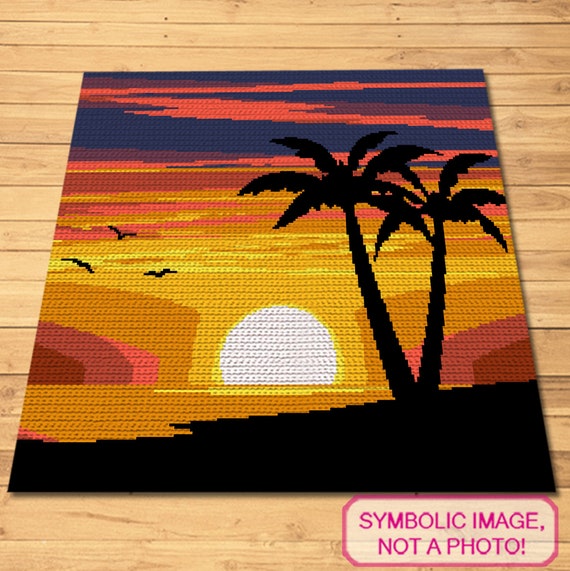The image depicts a detailed piece of art, likely created through crochet or another textile medium, positioned on a wooden floor made of slats. The artwork illustrates a vibrant sunset or sunrise, characterized by a series of colors transitioning from light yellow and gold near the horizon to pinks, reds, and maroons in the sky. At the center, the sun is depicted in white with an orange outline, casting its glow on the water below, which is a mix of orange and pink.

To the right of the sun, two black silhouetted palm trees stand on the shore, and to the left, three black birds—likely seagulls—are seen flying. The sky features horizontal bands of pink clouds against varying shades of a blue to golden backdrop, creating a dramatic and layered visual effect.

The bottom right corner of the artwork contains a rectangular text box outlined in pink with a white interior, clearly stating, "symbolic image, not a photo," indicating that this piece is a generated or representative image rather than a photograph. The art piece as a whole showcases intricate details and a rich palette, capturing the serene beauty of a coastal sunset or sunrise.